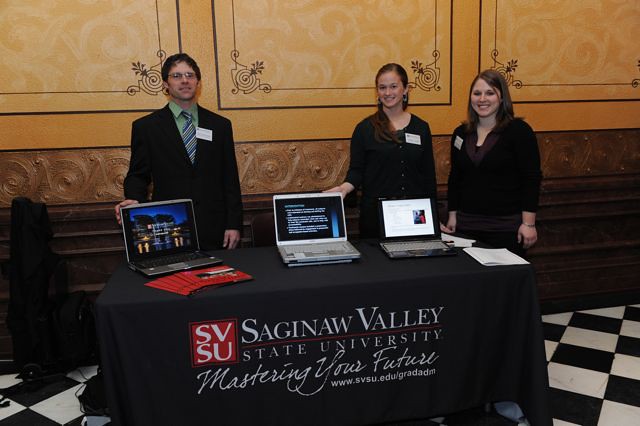This indoor photo features three young professionals, two women and one man, standing behind a display table draped with a black cloth that reads "Saginaw Valley State University, Mastering Your Future" along with the website "www.svsu.edu/gradadm." To the left, the man is a Caucasian male dressed in a black suit paired with a green dress shirt and a colorfully designed diagonally striped tie. He sports glasses and has medium-short hair, along with a white name badge pinned to his suit. His hand rests on a black laptop. Standing beside him are two Caucasian women, both with long brown hair and dressed in all black. Each woman is positioned beside an open laptop; the woman next to the man has her hand on a silver laptop, while the other laptop sits next to additional materials on the table. The table also holds white sheets of paper and shiny red pamphlets resembling little magazines. Both women wear name tags, and one of them has a bracelet on her left arm. The trio is smiling, contributing to the engaging and professional atmosphere of the scene.